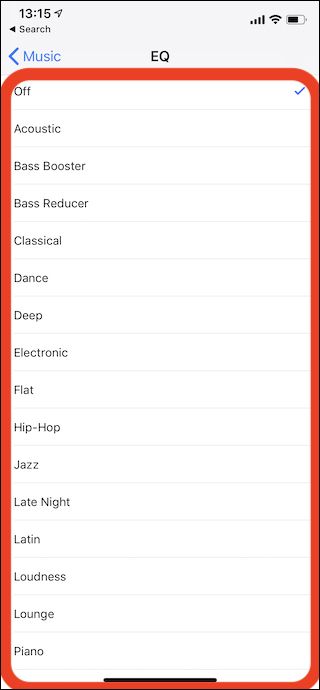The image depicts a detailed interface of a cell phone screen displaying the music equalizer (EQ) settings. At the top, the time is shown as 13:15, accompanied by indicators for cell phone signal strength, Wi-Fi, and battery status. Below these indicators, there is a search icon and a left-arrow button, suggesting a navigational option. 

Centered at the top of the screen is the title "EQ," indicating the equalizer settings. The main section of the screen consists of a vertical list of various EQ presets on the left side, each circled by a thick red rectangle with rounded corners. The presets are organized in the following order from top to bottom: "Off," "Acoustic," "Bass Booster," "Bass Reducer," "Classical," "Dance," "Deep," "Electronic," "Flat," "Hip Hop," "Jazz," "Late Night," "Latin," "Loudness," "Lounge," and "Piano." Each preset is separated by a horizontal gray line extending across the screen from left to right. 

Currently, the "Off" preset is selected, indicated by a blue check mark. The bottom of the screen features a black line just beneath the red outlined area. The screen mainly uses a color palette consisting of white, black, blue, and red.